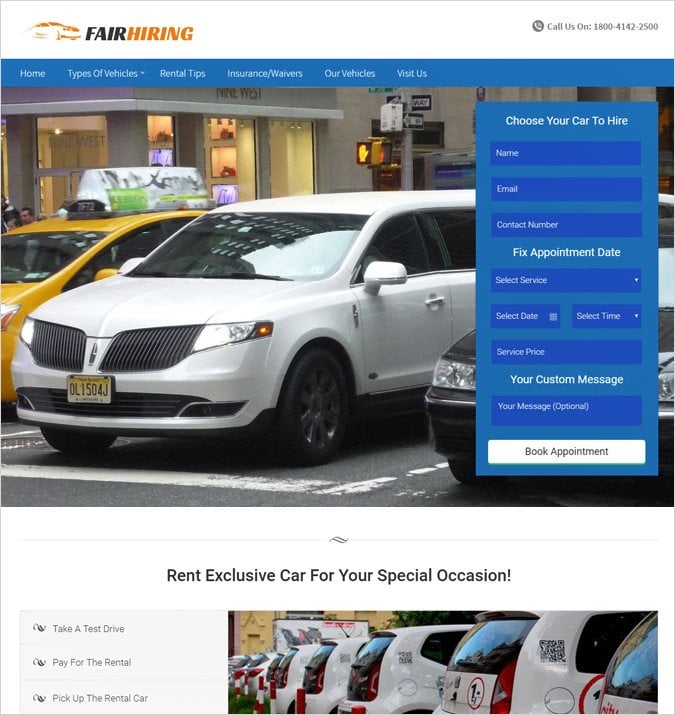In the vibrant scene depicted in the image, a bustling car rental advertisement showcases a variety of vehicles, including a yellow taxi, a white limousine, and a sleek black car, all positioned in front of a modern building adorned with a "West" sign. The image conveys the availability of diverse rental options, highlighted by an organized interface displayed within a prominent blue rectangle on the side.

The detailed interface invites users to "Choose Your Car to Hire," prompting them with boxes to enter their name, email, contact number, and other essential details such as appointment date and time, service price, and custom messages. Additionally, action prompts like "Book Appointment" and "Rent Exclusive Car for Your Special Occasion" are neatly arranged within the white rectangles for easy navigation.

A row of pristine white vans is lined up, emphasizing the company's extensive fleet, ready for test drives or rentals. Key services are outlined, including home vehicle types, rental trips, insurance/waivers, and the simplicity of the rental process with clear steps: "Take a Test Drive," "Pay for the Rental," and "Pick Up the Rental Car." 

The image is complete with a visually appealing mix of orange and black branding elements and a contact number, 1-800-414-2500, ensuring accessibility and convenience for potential clients.